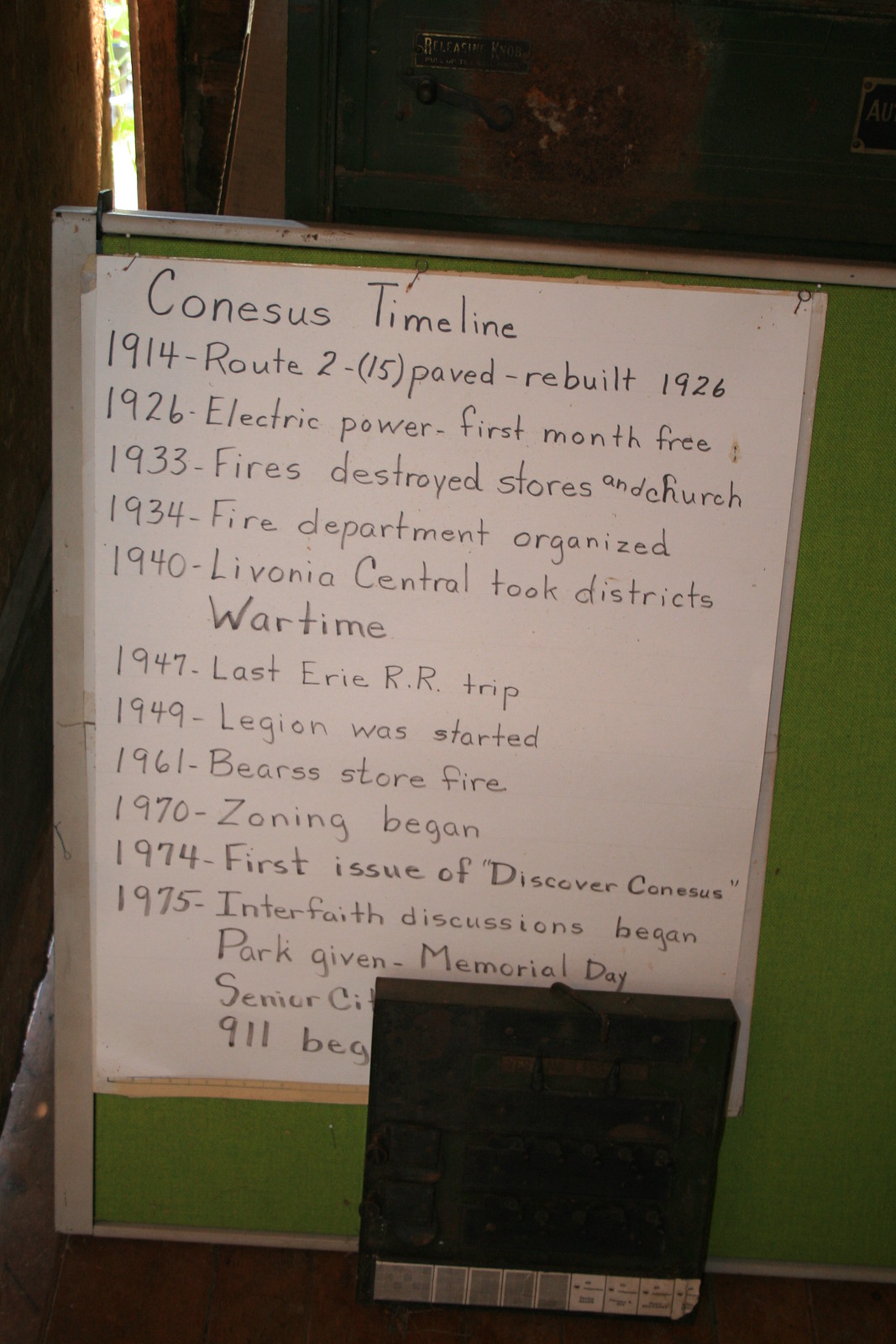The image showcases a close-up of a green bulletin board with silver trim and tan edges. Positioned prominently on this board is a large white piece of paper titled "Conesus Timeline," written in pencil. The timeline lists several historical events and corresponding dates:

- 1914: Route 2 Paved, Rebuilt 1926
- 1926: Electric Power, First Month Free
- 1933: Fires Destroyed Stores and Church
- 1934: Fire Department Organized
- 1940: Livonia Central Took Districts Wartime
- 1947: Last Erie Railroad Trip
- 1949: Legion was Started
- 1961: Bears Store Fire
- 1970: Zoning Began
- 1974: First Issue of Discover Conesus
- 1975: Interfaith Discussions Began, Part Given Memorial Day

A black, square-shaped recording device with a light-colored band and possibly barcodes sits in the front, partially obstructing the bottom right-hand side of the paper. Behind the green board, there's a barely visible window with drapes on the left side, casting a shadowy background.